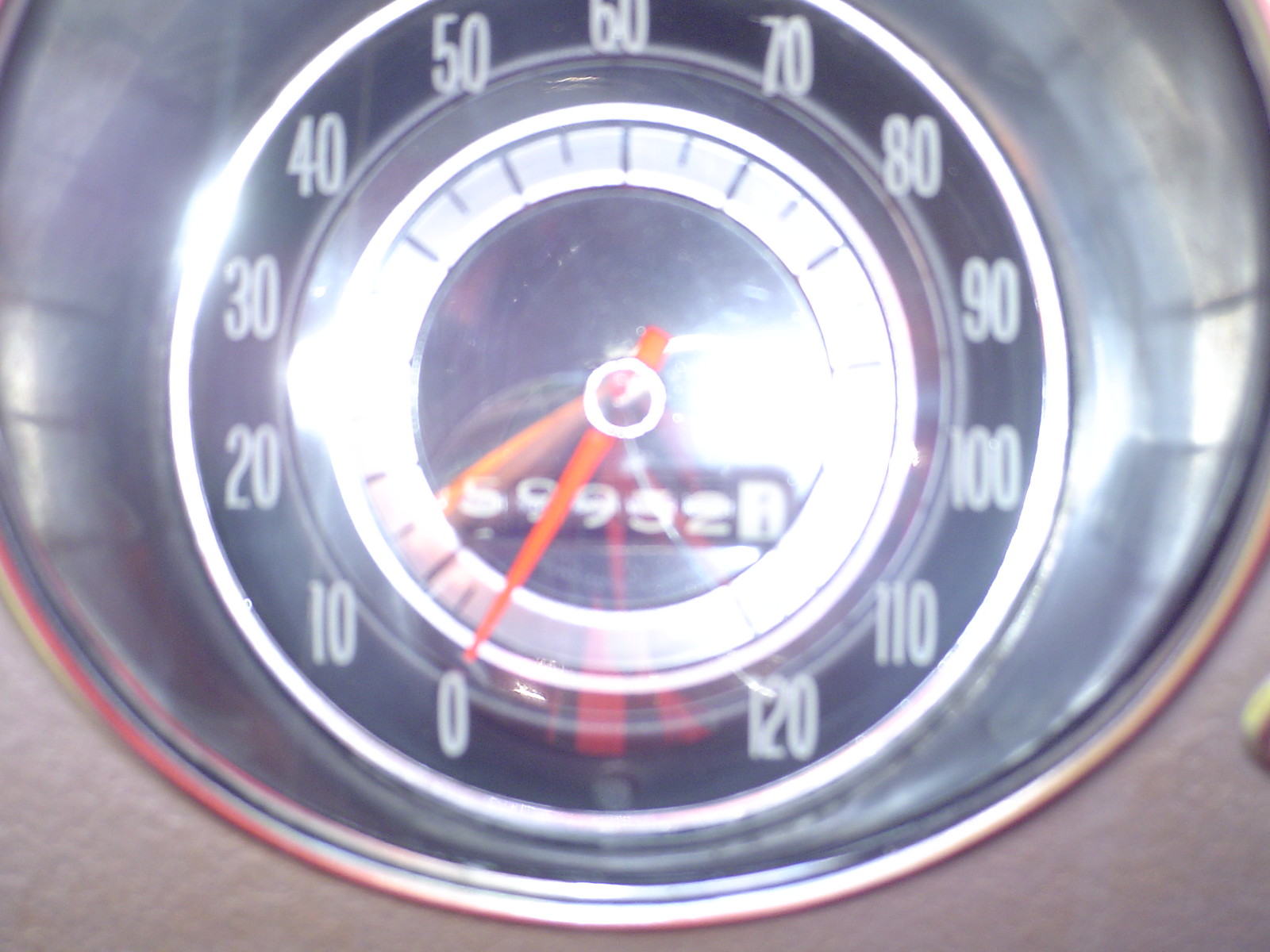This image captures a speedometer, framed by two triangular, brown sections at the bottom left and right corners, reminiscent of wall textures. The focal point of the photograph is the speedometer itself, which is zoomed in and slightly blurry.

Encircling the speedometer is a metal band with a reddish hue. The interior of the speedometer features a black face. Central to this black area is a circular section where the numbers are displayed. The numbering begins at 0 on the left side and increases incrementally clockwise: 10, 20, 30, 40, 50, 60, 70, 80, 90, 100, 110, and finally 120.

Within the center, there is a smaller black circle that houses the numbers. From this circle, an orange needle extends, currently pointing to 0. Beneath the needle, the odometer reads 59952 with an indistinct final digit, possibly an 8. There is a noticeable light reflection in the middle of the image, accompanied by a faint reflection of a person in the upper left corner of the speedometer's glass cover. The outermost part of the speedometer appears to be made of glass.